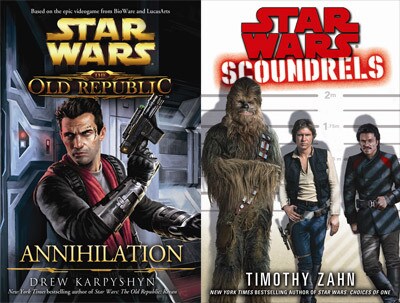The image showcases two book covers side by side, both pertaining to the Star Wars universe. 

The left cover features a vividly illustrated digital painting with the title "Star Wars: The Old Republic - Annihilation" in prominent gold text at the top, using the iconic Star Wars font, and subtitled "Annihilation" in matching gold and white text at the bottom. The author, Drew Karpyshyn, is noted below in small, white text. The art depicts a man with brown hair dressed in a black jacket, black gloves, a red scarf, and a gray shirt, holding a futuristic black laser gun, standing inside what appears to be a spaceship.

The right cover, in contrast, presents a lineup-style illustration with three well-known characters from the original Star Wars movies, standing against a background marked with height lines, resembling a police lineup. Chewbacca is on the left, with Han Solo and another man believed to be Luke Skywalker on the right. The title features "Star Wars" in a bold red logo at the top, with "Scoundrels" below it in white stencil-styled lettering that appears spray-painted. The author, Timothy Zahn, is credited at the bottom.

The detailed renditions of both covers highlight contrasting themes: a stark, singular character moment in a futuristic setting on the left, and a nostalgic, character-driven scene on the right, linking both to the rich Star Wars narrative.